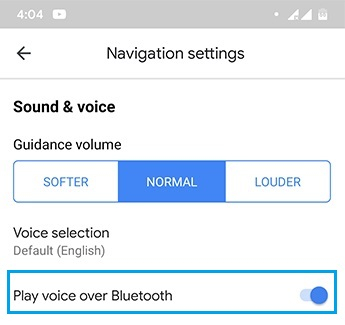This is a detailed screenshot of a website captured from a smartphone, displaying the top half of the phone's screen.

At the top of the image, there is a light gray status bar. On the left side of this bar, there is a "404" error code, and next to it is a YouTube icon. On the right side, there is a dot followed by a signal bar icon, which indicates a fully filled signal strength with two bars, one of which has a small square on its corner. At the very right edge of the status bar, there is another icon that is not clearly identifiable.

Below the status bar, on the left-hand side, there is a left-pointing arrow. Centered beneath the arrow, the text "Navigation settings" is prominently displayed. A gray line separates this section from the next content block.

The subsequent section starts with the bolded title "Sound and voice." Directly beneath this heading, the text "Guidance volume" is present. Following this, a rectangular slider is divided into three labeled sections: "Softer" on the left, "Normal" in the center (highlighted with a blue background), and "Louder" on the right (both "Softer" and "Louder" have a white background similar to the surrounding area).

Lower on the page, another bolded heading reads "Voice selection." Below this heading, it states "Default (English)" indicating the chosen language setting. Further down, there is an option titled "Play voice over Bluetooth," which features a toggle switch currently turned on. This toggle is accompanied by a rectangle bordered in blue.